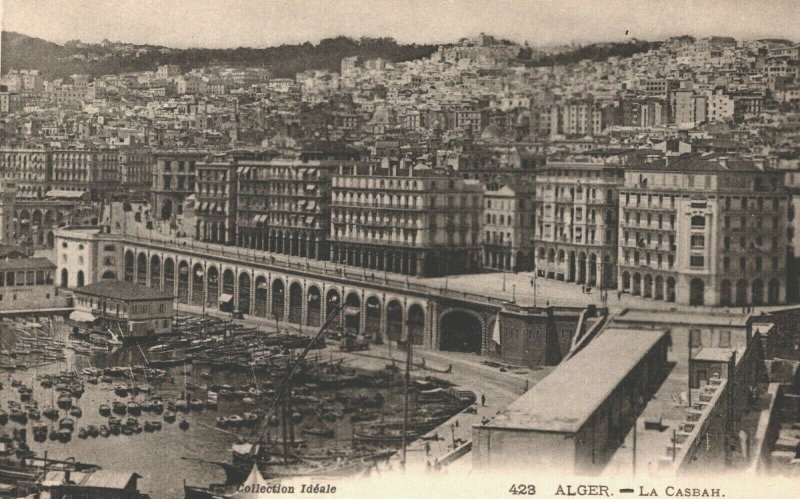This antique black and white postcard features a detailed depiction of a historic port city, likely somewhere in French-speaking North Africa, as evidenced by the text at the bottom that reads "Collection IDÉALE EDL" and "423 Alger ALGER-LACASBAH." 

The image captures a bustling harbor situated in the bottom left corner, filled with an array of docked boats. Behind the harbor lies a bridge that connects the waterfront to a sprawling urban settlement. 

The cityscape is dominated by numerous multi-story buildings, which appear to be a mix of apartment complexes and houses, characterized by their abundant windows and doors arranged in orderly rows. These structures ascend the hillside in a grand, repetitive fashion, evoking a sense of architectural uniformity and grandeur.

As the buildings climb higher up the mountain, they gradually diminish in size, eventually blending into the rugged mountain terrain in the background. This photographic scene is rendered even more nostalgic by its black and white, grayscale palette, and the visible signs of aging, including scratch marks and faded patches, which enhance the historical charm of the postcard.